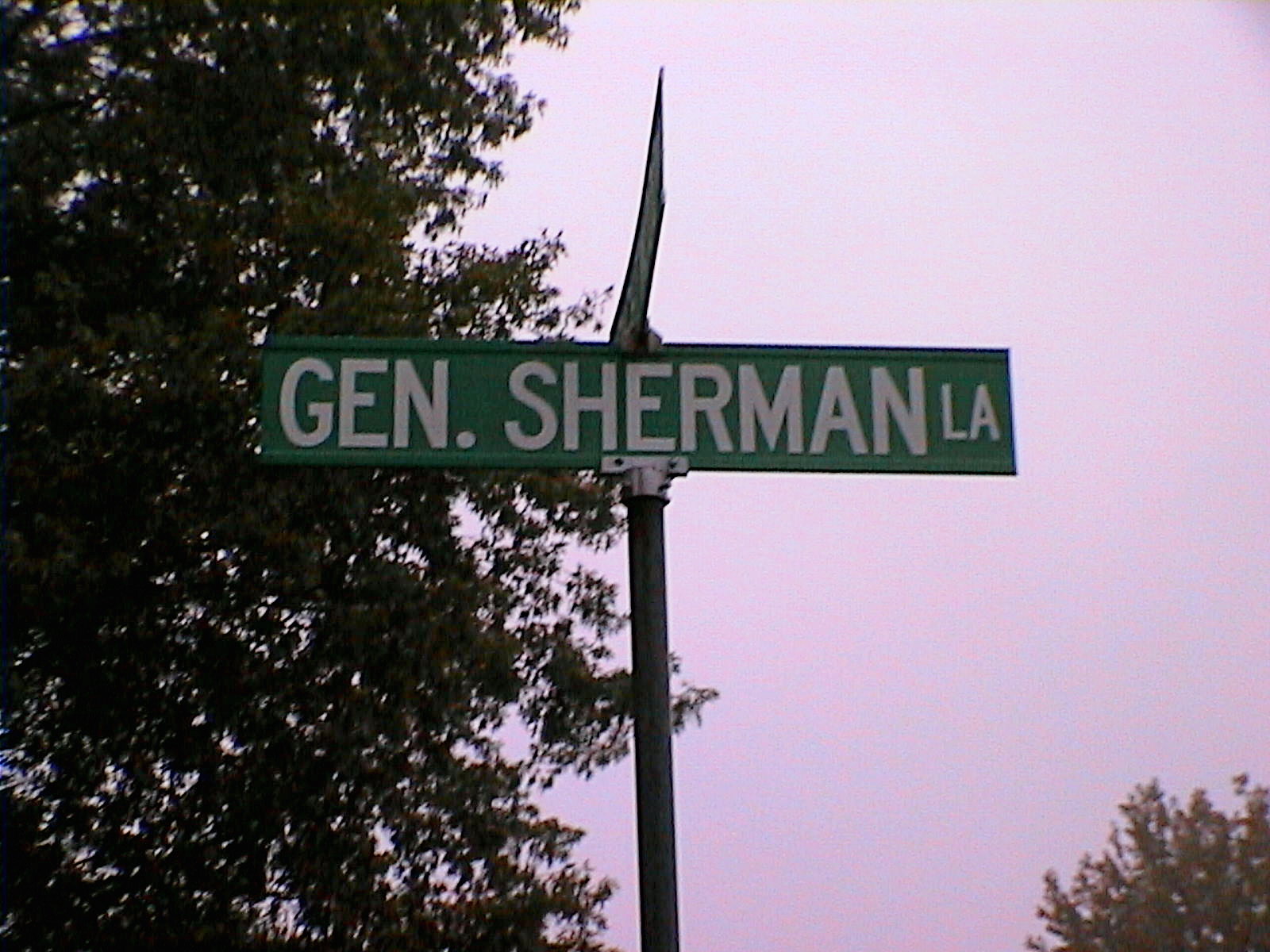The rectangular photograph prominently features a street sign reading "GEN. SHERMAN LA," situated on a black pole. This green, rectangular sign, approximately six inches in length and an inch and a half in height, is displayed in white capital letters. The image is captured from a lower angle, looking up at the sign, giving a slight sense of elevation. An additional sign for another street, facing the opposite direction, is mounted atop it but remains unreadable from this perspective.

The background sky spans across the right side of the image, presenting a light pink hue indicative of overcast conditions. On the left side, a large, green-leaved tree is visible, occupying nearly half of the image. Another tree, blurred and less distinct, is faintly visible in the lower right corner. Both trees frame the photograph, enhancing the natural setting surrounding the street sign.